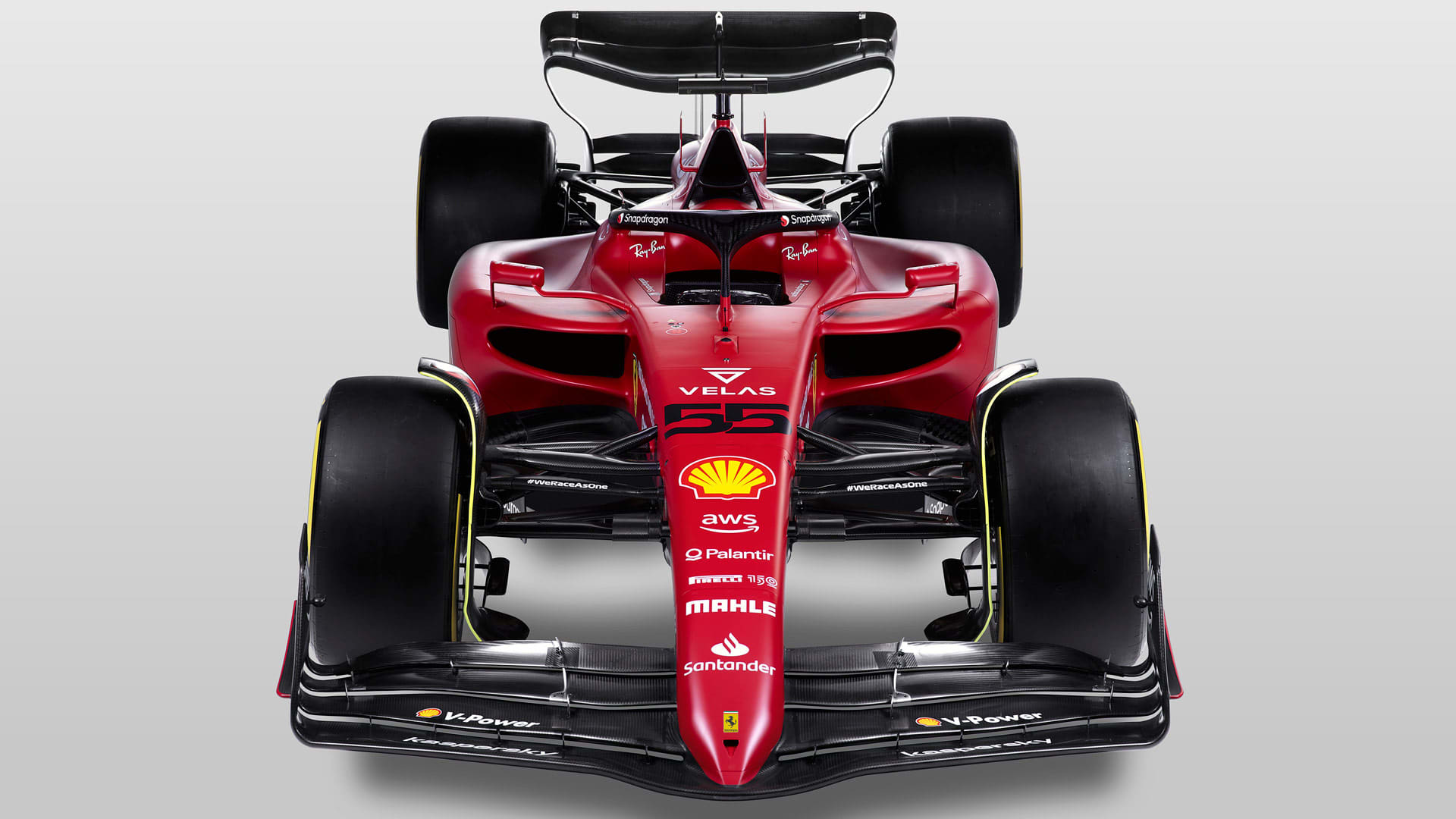The image depicts a striking Formula One race car, positioned centrally against a completely light gray background. The car is oriented with its front end facing directly towards the viewer. Notably, the car's body is predominantly red, accented with various logos and advertisements. The prominent Shell logo is displayed on the front, along with other brands including Santander, AWS, Palantir, and Mahle. The number 55 is also visible, as well as a logo that says "VELAS" in silver, featuring an upside-down triangle design.

The car lacks a hood and a top, giving it a sleek, open-wheel appearance. Its narrow front end, reminiscent of the letter "V," features a black grill or protrusion hanging down the middle. Each side of the front top section is adorned with mirrors. The bumper is black and displays "V-Power" on each side, while the slick, flat tires are fully visible, emphasizing their large, sturdy design. At the rear, a tall black spoiler extends upwards, contributing to the aerodynamic structure of the race car. Additionally, the hashtag "WeRaces1" can be spotted amongst the detailed writing on the vehicle.